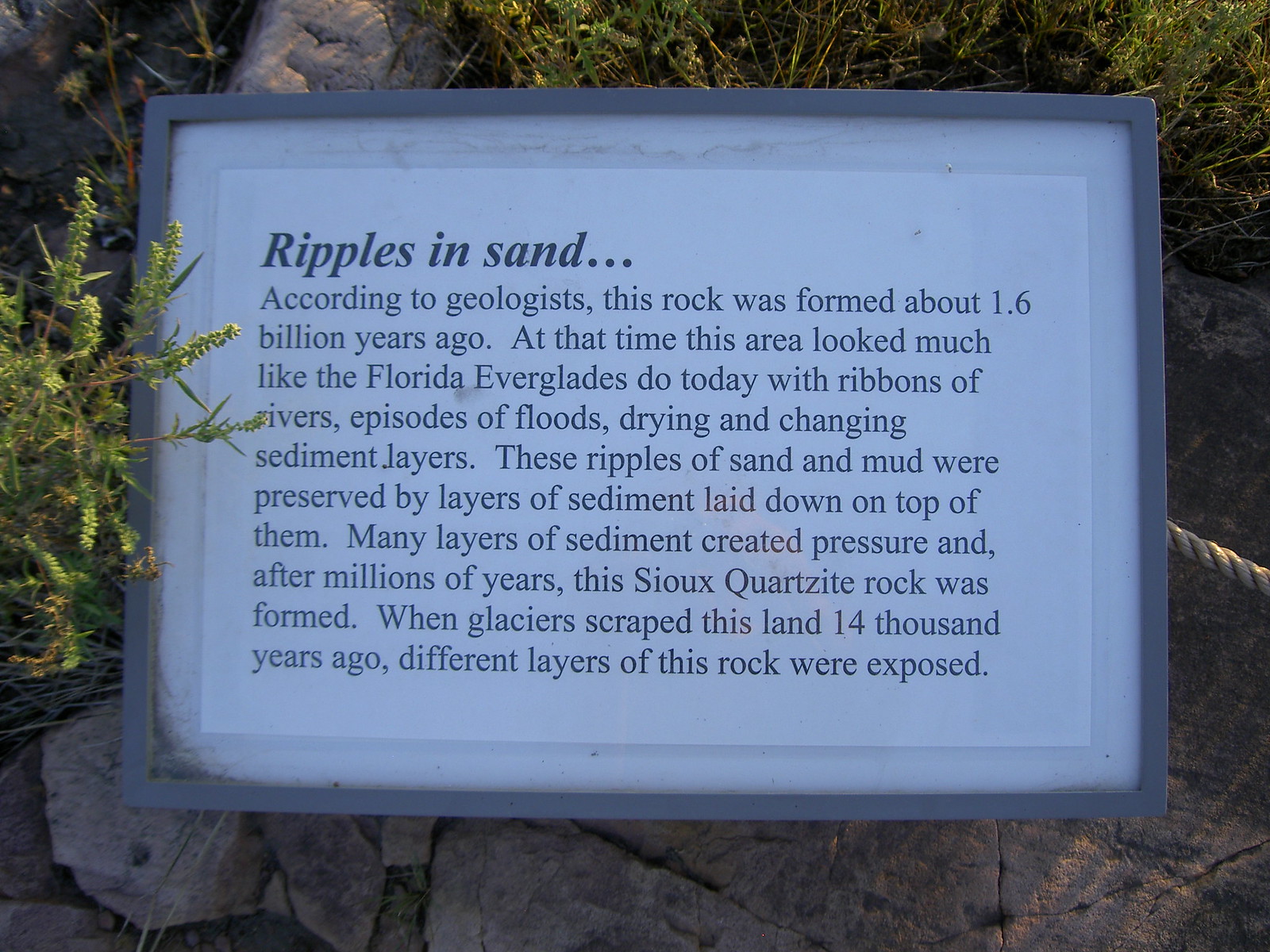The image captures a close-up view of a framed informational plaque in an outdoor setting. The plaque, encased in a dark gray metal frame, looks like a piece of paper inside a clear glass frame. The plaque, positioned horizontally, bears the large, bold italicized headline "Ripples in the Sand…" beneath which the text reads: "According to geologists, this rock was formed about 1.6 billion years ago. At that time, this area looked much like the Florida Everglades do today, with ribbons of rivers, episodes of floods, drying and changing sediment layers. These ripples of sand and mud were preserved by layers of sediment laid down on top of them. Many layers of sediment created pressure, and after millions of years, the Sioux Quartzite rock was formed. When glaciers scraped this land 14,000 years ago, different layers of this rock were exposed." The plaque is situated against large stones and surrounded by a natural setting of rocks, leaves, and grass. A faint silhouette of the photographer is faintly visible, reflected in the glass on the center-right. A piece of rope is seen extending from the center-right of the image, seemingly securing the plaque in place.